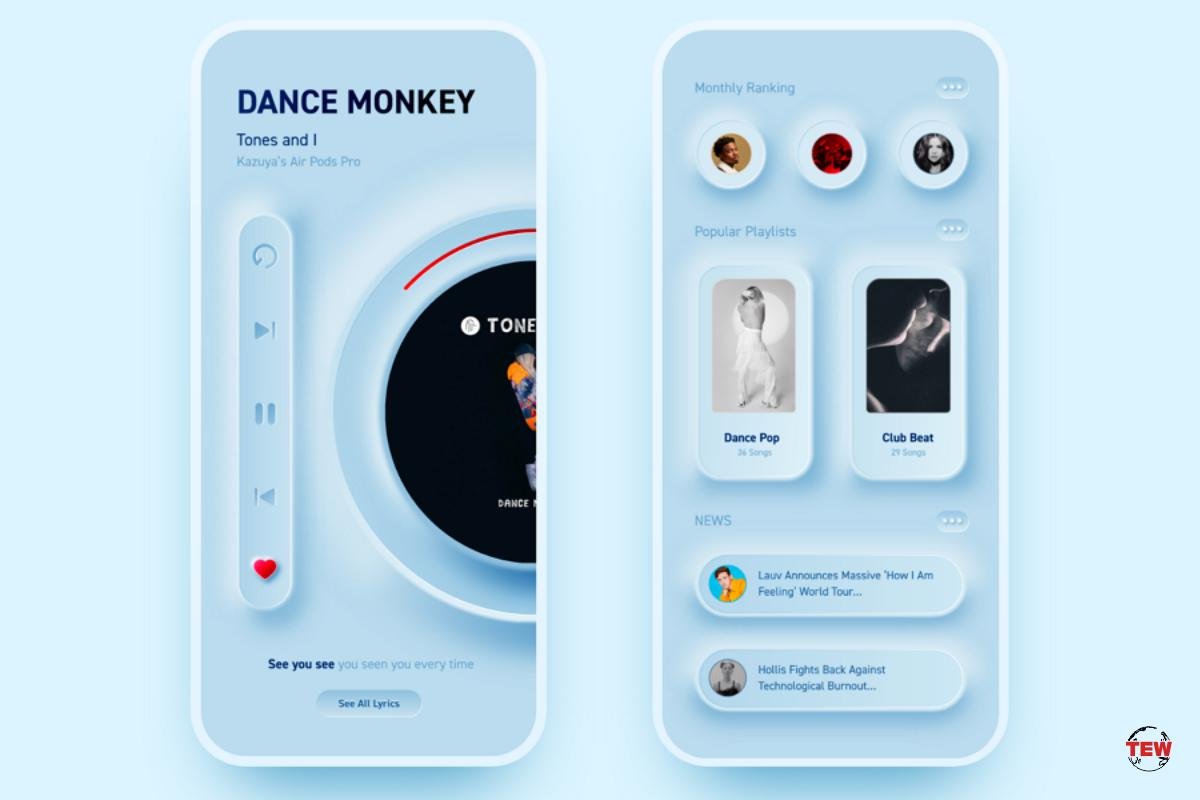The image showcases a close-up of two identical white iPhones positioned side-by-side against a light blue background with a red "TEW" logo featuring a globe in the bottom right corner. The phone on the left displays a music app screen with "Dance Monkey" by Tones and I, paired with the phrase "Kazooia's AirPods Pro." Below this title, the screen features various music control icons including play, pause, rewind, and heart buttons. There is also a partial view of an album artwork circle.

The phone on the right highlights a different section of the app, beginning with a "Monthly Ranking" heading and three circular profile pictures of artists. Below this, there are rectangular sections labeled "Popular Playlists" with titles such as "Dance Pop" and "Club Beat." The bottom portion of this screen lists "News" with snippets of music-related headlines.